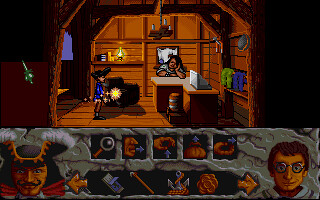This vibrant color image depicts an engaging scene from a video game, likely from a computer or console platform. The upper portion of the scene showcases a cozy cabin room, characterized by its warm brown walls and rustic interior. A window is prominently situated on the left-hand side, accompanied by various pieces of wooden furniture that add to the room's homely atmosphere. Mounted on the wall shelf is a lit lamp, casting a gentle glow over the surroundings.

In the left-hand corner of the cabin stands a small character, identifiable by their blue top, facing right. Nearby, countertops are adorned with objects, including a noticeable white item. The right-hand wall features hanging blue and green objects, adding a touch of color and intrigue to the scene. A notable green sword lies on the left, hinting at potential adventure or combat elements within the game.

The lower part of the image transitions into a control interface, presumably for gameplay management. This area is flanked on either side by distinctive character faces: the left side features a face with horn-like protrusions or an unusual head shape, while the right side displays a bespectacled male or boy. Central to the interface are small squares filled with infographics, though their details are indiscernible.

Overall, the image blends nostalgic charm with the excitement of exploration and interaction, typical of a well-crafted video game environment.